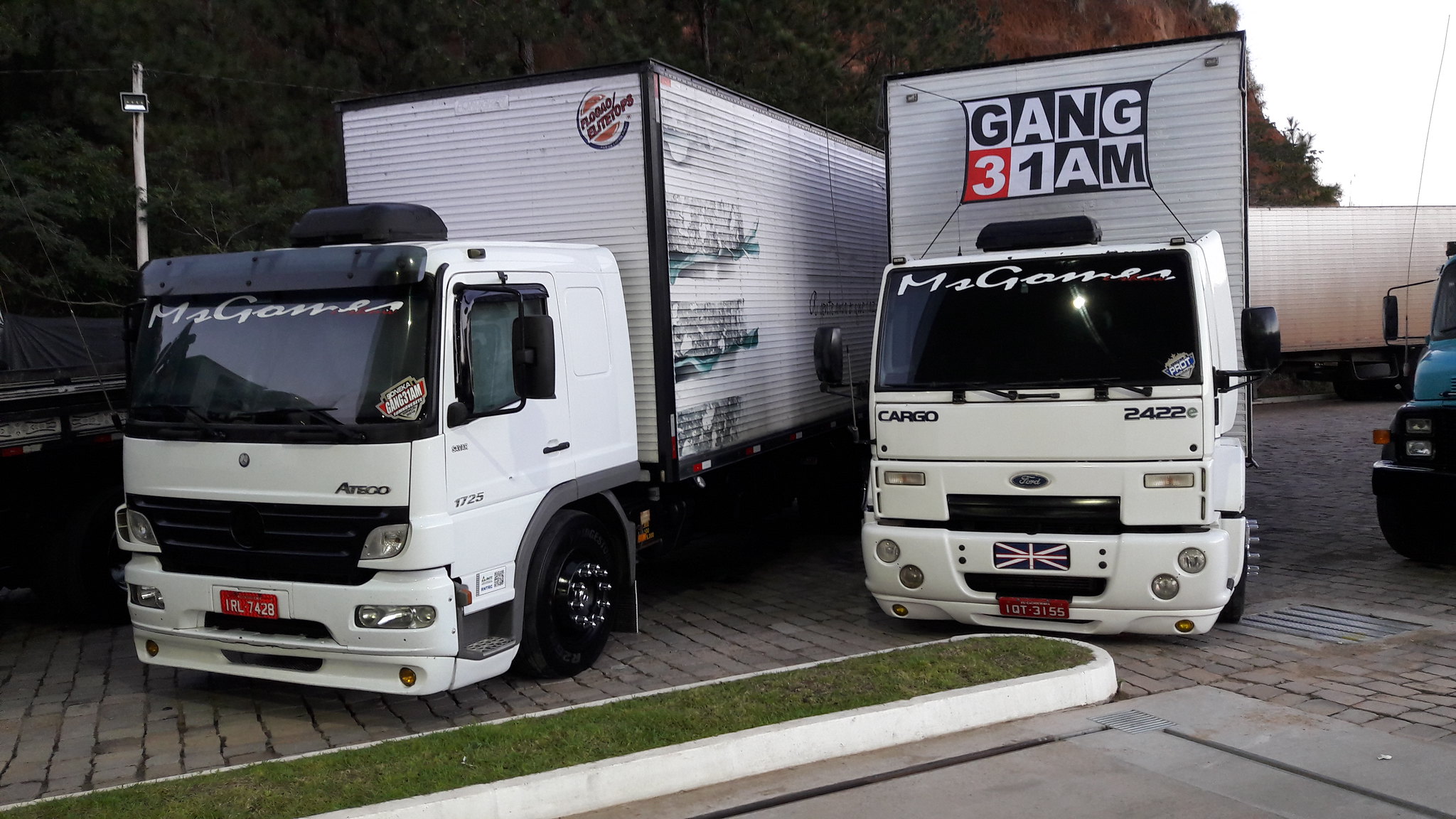The image is a horizontally oriented color photograph featuring two prominently visible white trucks with black tops, standing on a cobblestone walkway. The trucks, which may be 18-wheelers, have tinted windows and white text on the front windshields, possibly reading "Mr. Games" or "Miss Games." The truck on the right has the phrase "Gang 31 AM" displayed in a checkerboard pattern above the windshield, with the numeral 3 in white text on a red background. Both trucks are positioned near a strip of grass bordered by a white cement curb that extends from the left side toward the right-hand side at the bottom of the image. In the lower right corner, there is a metal grate beside another portion of the curb or sidewalk. A possible third truck, appearing blue or greenish-blue, is barely visible to the right. The background includes grassy fields, enhancing the outdoor setting. Additionally, a detail of a British flag is located where a license plate would typically be on one of the trucks.